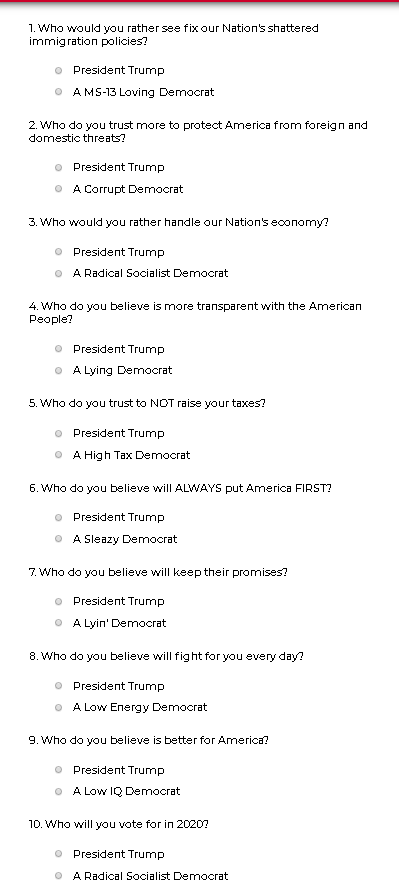This is a screenshot of a politically charged survey designed to capture respondents' opinions on various issues. The survey comprises ten questions, each comparing President Trump with a derogatorily described Democrat. The visual presentation is quite plain, featuring a white background and black text, with a thin red banner spanning the top. Each question offers only two possible responses. The questions are as follows:

1. Who would you rather see fix our nation's shattered immigration policies? 
  - President Trump 
  - MS-13 loving Democrat

2. Who do you trust more to protect America from foreign and domestic threats?
  - President Trump
  - Corrupt Democrat

3. Who would you rather handle our nation's economy?
  - President Trump
  - Radical Socialist Democrat

4. Who do you believe is more transparent with the American people?
  - President Trump
  - Lying Democrat

5. Who do you trust to not raise your taxes?
  - President Trump
  - High Tax Democrat

6. Who do you believe will always put America first?
  - President Trump
  - Sleazy Democrat

7. Who do you believe will keep their promises?
  - President Trump
  - Lying Democrat

8. Who do you believe will fight for you every day?
  - President Trump
  - Low Energy Democrat

9. Who do you believe is better for America?
  - President Trump
  - Low IQ Democrat

10. Who will you vote for in 2020?
  - President Trump
  - Radical Socialist Democrat

The language used in the survey is overtly biased, frequently employing pejorative terms to describe the Democratic options, suggesting an attempt to influence the perspectives of the respondents.